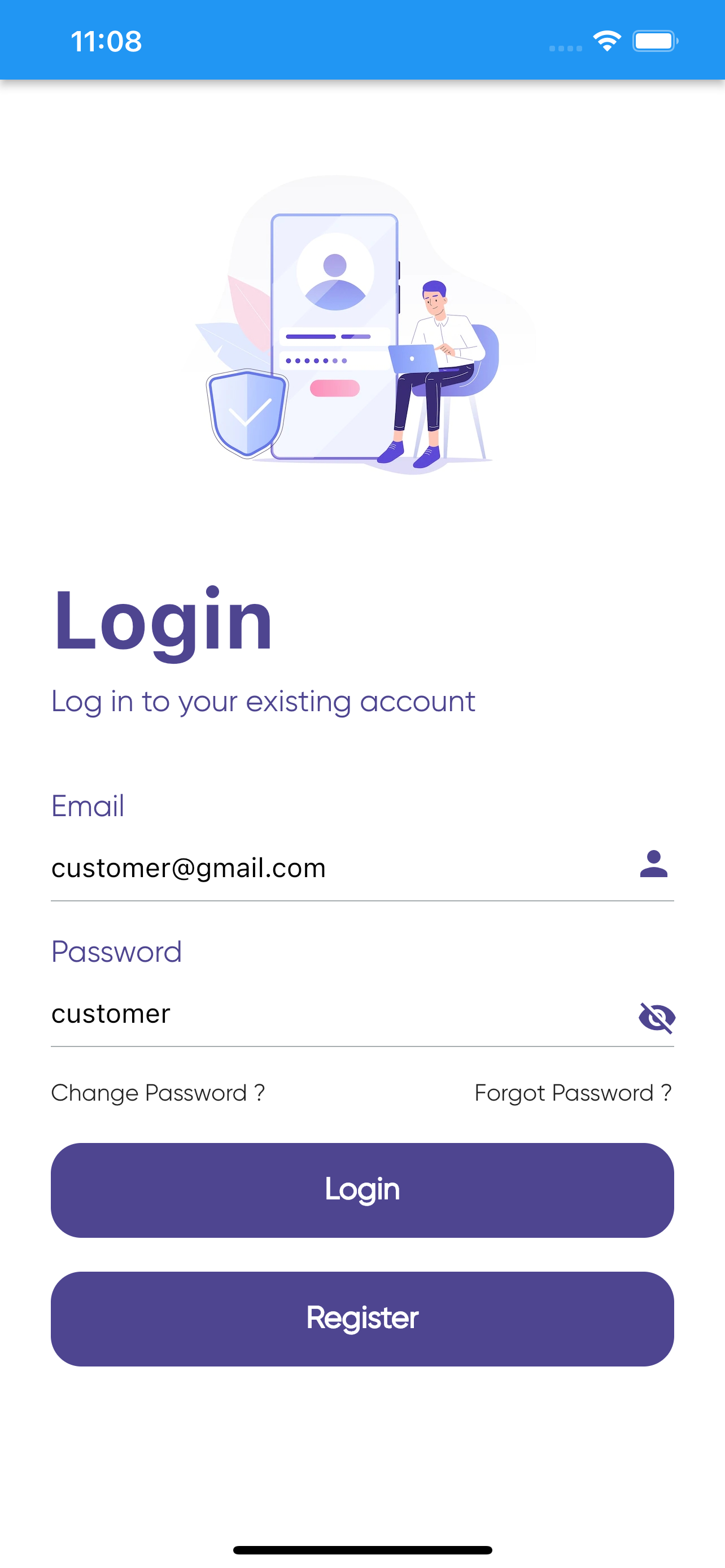The screenshot showcases a login screen on a smartphone. The top blue header displays the current time, 11:08 AM, followed by four signal dots, a Wi-Fi icon, and a full 100% battery indicator. Below the header is an illustrated graphic featuring a man seated to the right with an open laptop, positioned to the right of a smartphone illustration. To the left of this setup is a shield icon with blue and pink leaves adorning the scene from the left side of the phone.

On the illustrated phone screen, there is a circular profile area containing a silhouette of a person, accompanied by a few dashed lines and dots with an unlabeled button beneath it, indicating a mock-up rather than a live app interface. 

Prominently displayed below the graphic, the word "Login" is seen in large purple letters, followed by the instruction "Login to your existing account." The "Email" field follows this, with a person icon positioned to the right. The email address "customer@gmail.com" is filled in black text, while all other text remains in purple.

Next, the "Password" field is displayed in purple, with the text "customer" underneath, shown in black and underlined. An eye icon with a line through it indicates that the password is hidden. Below these fields, there are options for "Change password?" and "Forgot password?" placed on the left and right respectively.

At the bottom, two large, wide buttons with rounded corners are aligned vertically; the top button is labeled "Login," and the bottom one says "Register." A black scroll bar is centered at the very bottom of the screen.